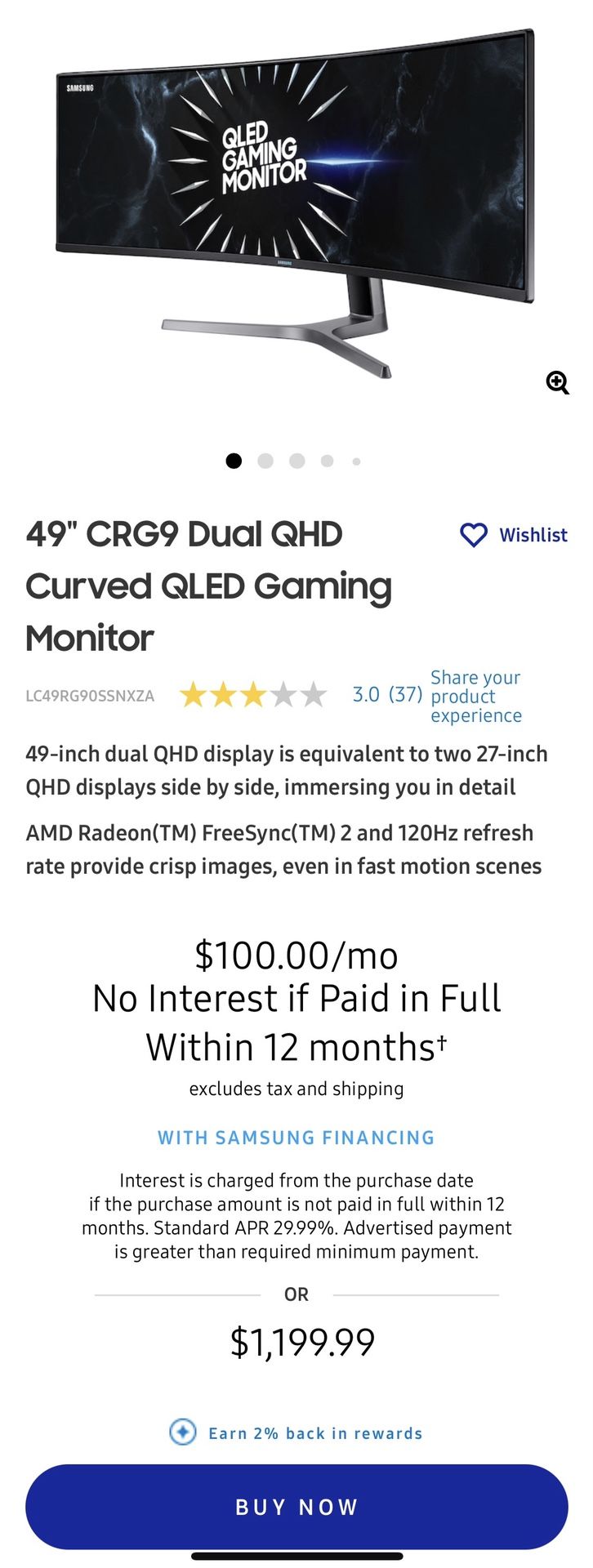This image showcases a sleek, curved gaming monitor prominently displayed at the top. The monitor is expansive, featuring a 49-inch screen with Dual QHD (5120x1440) resolution. In the center of the screen, "QLED Gaming Monitor" is emblazoned with radiating lines forming a circular design beneath the text. This visual element serves as an introduction to the monitor's standout feature. The full title "49-inch CRG9 Dual QHD Curved QLED Gaming Monitor" is presented below the image. 

The product has received a rating of three stars from 37 reviewers. Beneath the rating, a financing option is highlighted, stating: "$100 a month, no interest, if paid in full within 12 months." The total cost of the monitor is specified as $1,199.99. The detailed and polished presentation encapsulates the product's specifications, user feedback, and pricing options effectively.